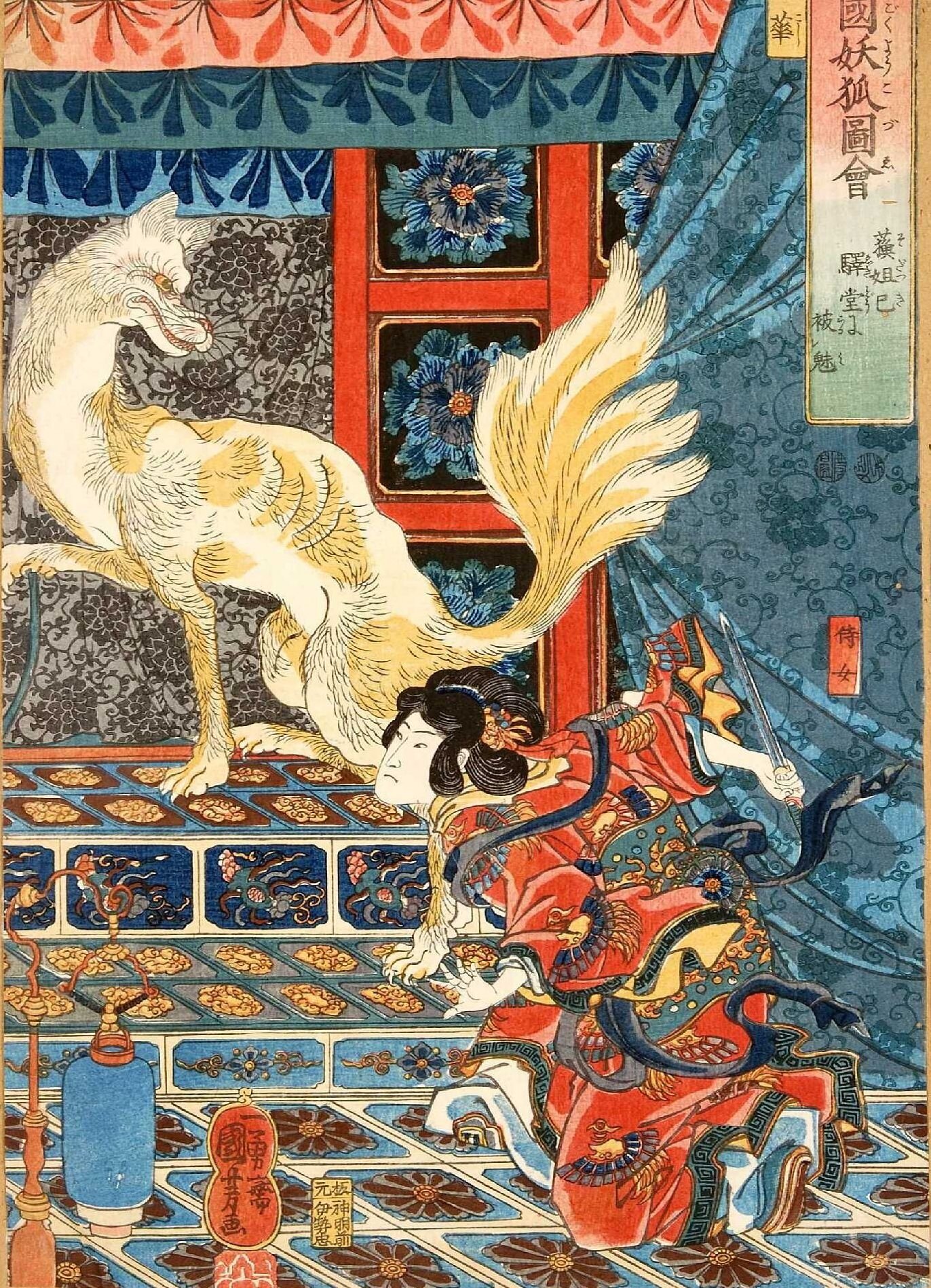The artwork in the image appears to be an intricately detailed, vibrant representation in an old Japanese style, possibly evoking a historical period. Dominated by rich hues of red, blue, and turquoise, the scene is set on a colorful, maroon-tiled floor patterned with floral motifs. A kneeling woman, dressed in a flowing red, blue, and turquoise kimono adorned with a dragon design, intensely gazes at a mythical creature. This creature, reminiscent of a multi-tailed fox or wolf, is depicted with yellow and white fur and possesses multiple tails emerging from its body, lending it an ethereal aura.

On the top right, a vertical sign adorned with oriental lettering adds to the scene's authenticity. The backdrop includes intricately painted banners and tapestries near the ceiling, brimming with floral designs, enhancing the overall illustrative quality typical of that period. Completing the picture is a blue jug on the floor, a red ladder, and various ornamental details that provide depth and context to this evocative, bohemian, and oriental image. The juxtaposition of the woman's serious expression and the fierce, mythical creature injects an intense narrative element into the artwork.